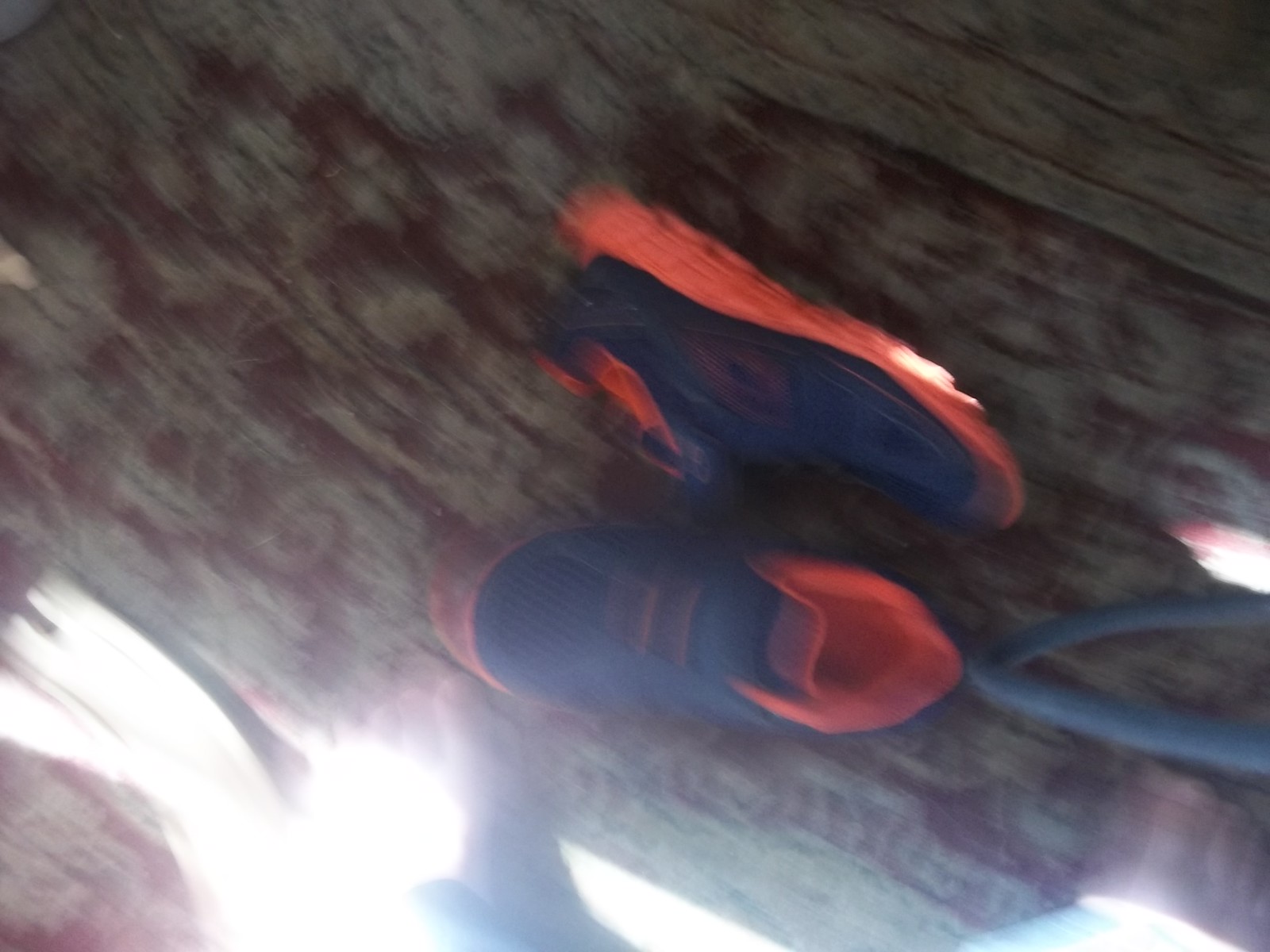The image portrays a very blurry photograph taken in an indoor setting, depicting a pair of athletic running shoes. One shoe lies on its side while the other stands upright. The shoes are primarily dark blue with neon orange interiors and soles, and the laces appear dark red. They rest on a dark red and possibly light brown rug with an intricate floral pattern, although there is some disagreement about the rug’s coloration, with another observation suggesting it could be green with a brown print. There is natural light overexposed at the bottom of the image, creating a stark contrast with the underexposed, darker upper part of the photograph. The feet of the person who took the photo are slightly visible, indicating that the image was captured with a personal camera.